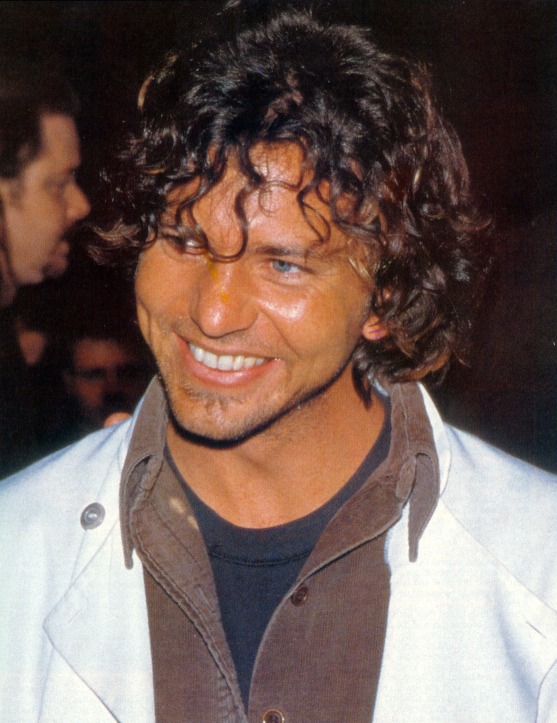This is a striking photo of Eddie Vedder, seen from the upper chest upward. Eddie, a handsome man with a medium, suntanned complexion, is smiling broadly, showcasing his very bright, white teeth. He has long, curly black hair that falls over his blue eyes. Eddie is dressed in a white jacket, which features a button or zipper on one side, over a brown corduroy button-down shirt that is open at the neck. Beneath the shirt, he wears a steel gray or navy t-shirt. The background is predominantly dark, but on Eddie's right side, the side profiles of two other men with dark hair can be seen. The first man is a Caucasian with a goatee facing forward, while the second man below him is blurry and indistinct. Eddie Vedder dominates the image, which is framed by a mostly black backdrop with minimal details.